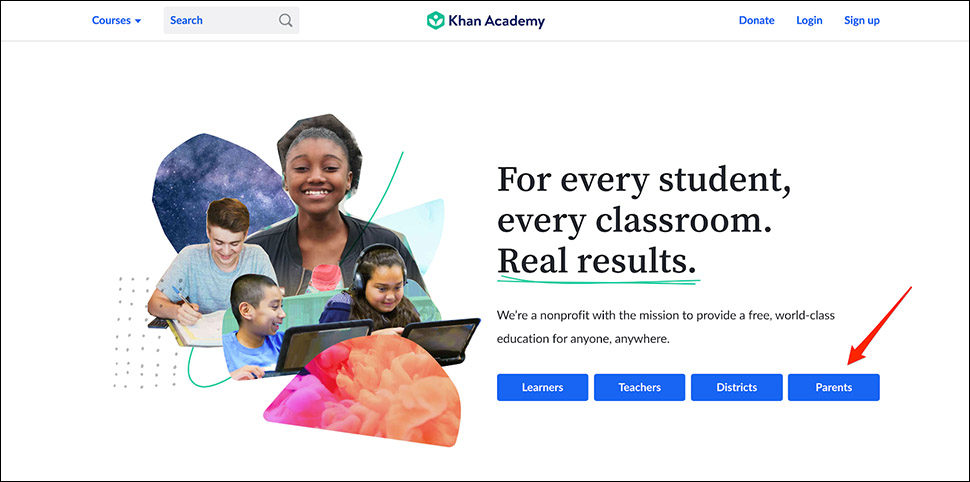The image is a captured screenshot of the homepage of the Khan Academy website. At the top of the page, "Khan Academy" is prominently displayed, indicating the organization's identity. The central area of the page highlights the mission statement: "For every student, every classroom. Real results." Below this aspirational message, the text elaborates, "We're a nonprofit with the mission to provide a free, world-class education for anyone, anywhere."

The layout of the site includes several navigational buttons designed to direct users to different parts of the website. These buttons are labeled: "Learners," "Teachers," "Districts," and "Parents." An arrow is specifically pointing towards the "Parents" button from the top, suggesting that the user might be guided to click there for further information or actions suitable for parents. The overall design is intuitive, with clear headings and an easy-to-follow navigational structure, aiming to support diverse educational needs.